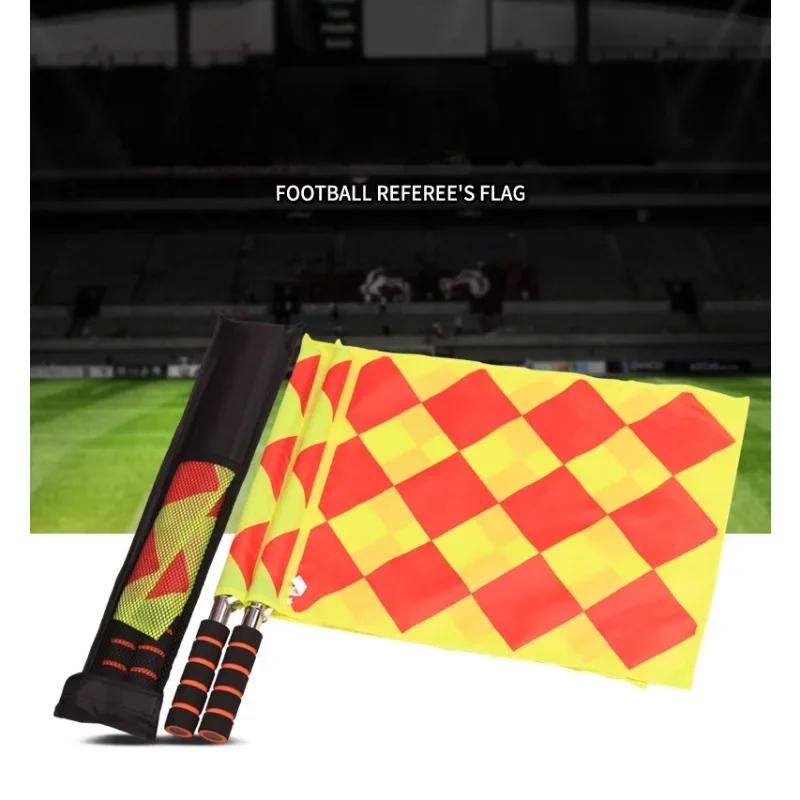The image is a detailed depiction of a football referee's flag presented in a layered format. The primary background is an empty football stadium with vivid green grass, but the stadium details are obscured by a dark opacity overlay. The text "Football Referee's Flag" is prominently displayed in white atop this darkened setting, ensuring high visibility. Superimposed on this background is the focal image of the referee's flag itself. The flag exhibits a distinctive checkered pattern, featuring neon yellow and neon red or pink squares arranged in alternating rows. The flag is affixed to a steel pole, which is fitted with a foam handle that has orange and black stripes for a secure grip. Accompanying the flag is a case positioned next to it, suggesting the storage or portability aspect of the equipment. The vibrant and professional design of the flag, along with the nuanced details of the handle and case, underscores its purpose and usability in officiating football games.